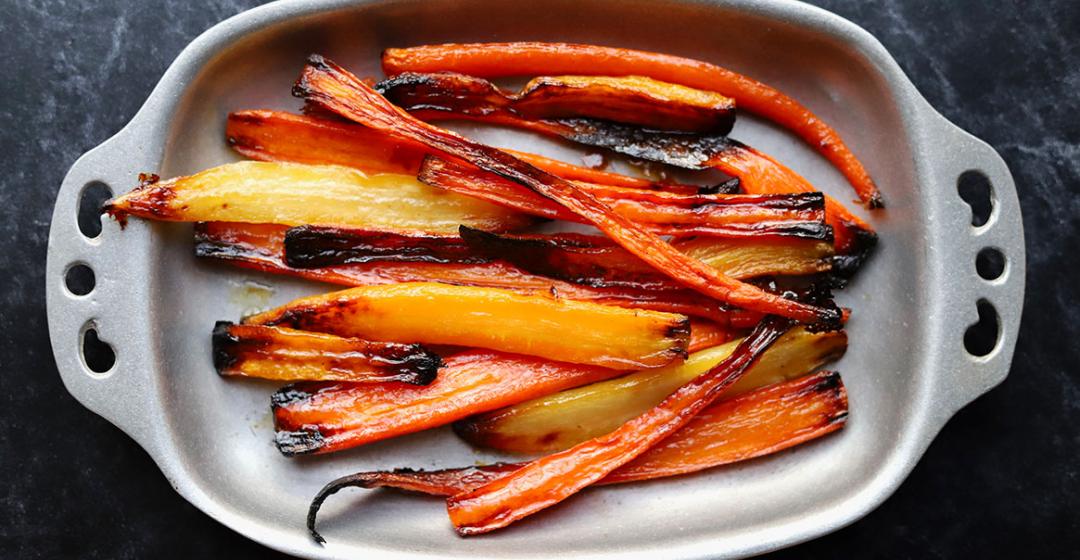The photograph captures a bird's-eye view of a rectangular, silverish ceramic dish placed on a marble-like black countertop. The dish, which features two handles each decorated with three holes (one round in the middle and two comma-shaped on either side pointing downward), contains an array of cooked vegetable strips, primarily carrots. The carrots vary in color from shades of yellow and orange to some blackened parts, indicating thorough cooking. They appear to be glazed in a brownish sauce, with some pieces slightly charred, giving them a grilled appearance. The vegetables are laid out in strips and slabs, totaling around 13 or 14 pieces of different shapes and colors within the oblong dish.